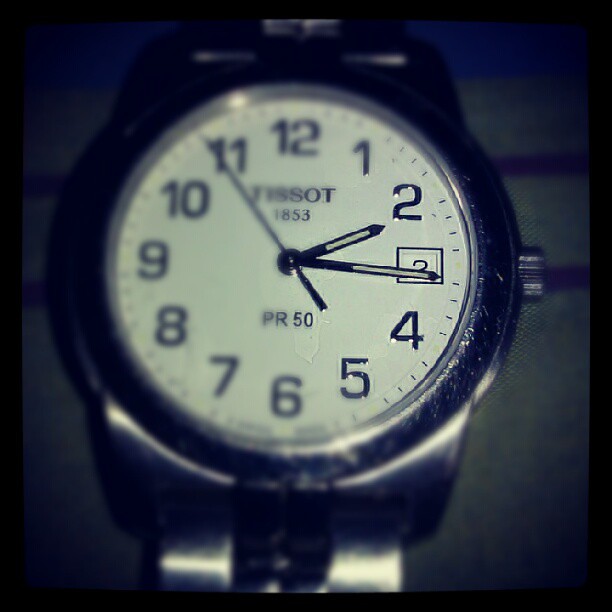This close-up photograph features a **Tissot 1853 PR 50 watch**. The timepiece, evidently well-worn, showcases numerous scratches on its silver metal casing, particularly around its bezel, indicative of extensive use. The watch's crown, used for adjusting time, is prominently visible on the right side. The face of the watch is white, marked with polished silver numerals and indices. The hands of the watch exhibit a unique design, with black extremities and partially translucent sections, while the slender second hand boasts a sleek silver hue. The dark grey background further accentuates the intricate details of the watch's face, offering a striking contrast and emphasizing its craftsmanship.